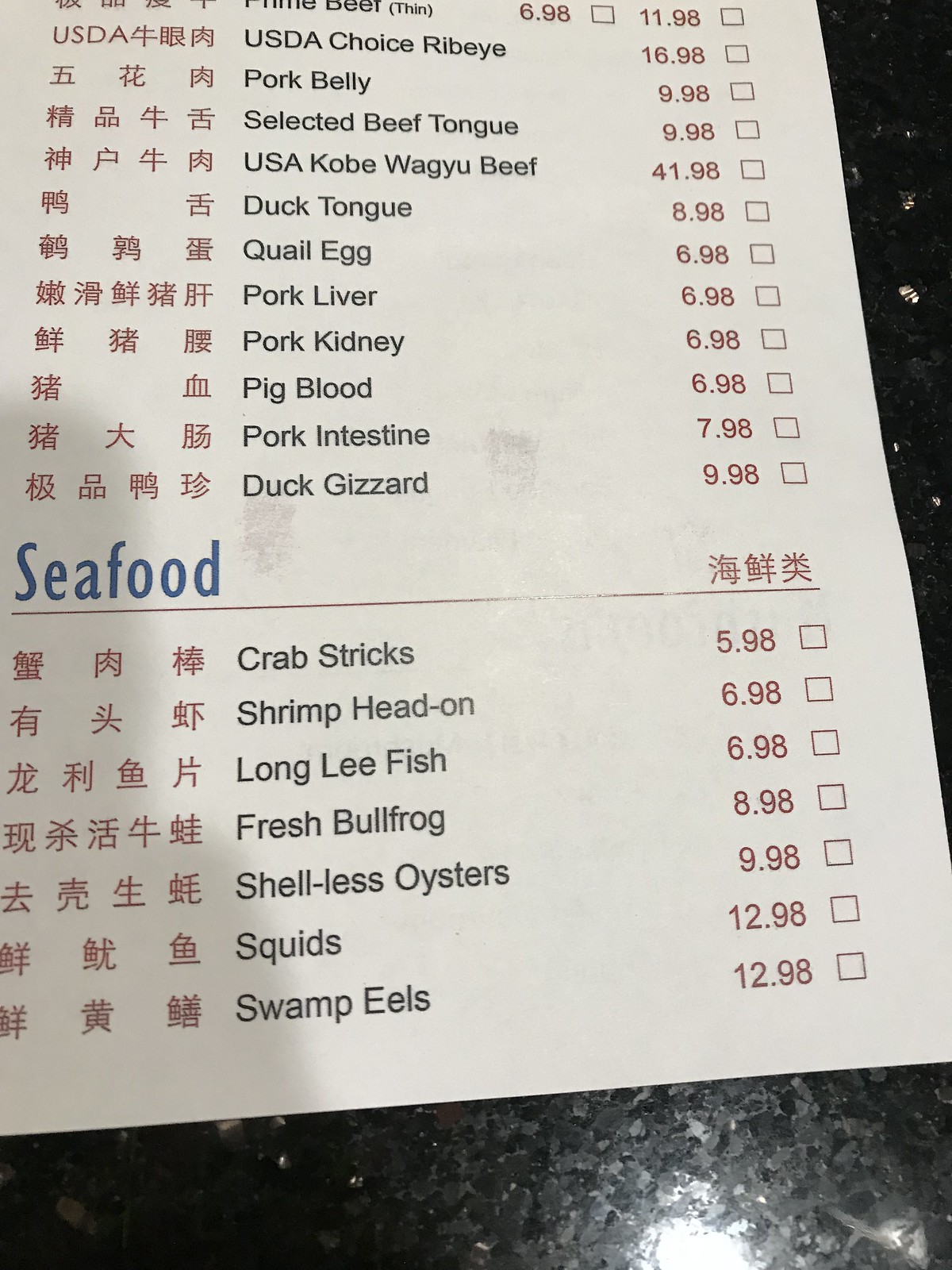This detailed image shows a neatly organized menu with various sections. On the left side of the menu, bold red text spells out "USDA," followed by "USDA Choice Ribeye" in bold black text. The price for this item, $16.98, is displayed beside it with a noticeable square marker.

The left-hand side of the menu is adorned with elegant Chinese calligraphy, adding an authentic touch. The menu items listed include an array of meats such as Pork Belly, Selected Beef Tongue, USA Kobe Wagyu Beef, Duck Tongue, Quail Egg, Pork Liver, Pork Kidney, Pig Blood, Pork Intestine, and Duck Gizzard.

Moving to the next category, "Seafood," and still accompanied by Chinese writing on the left, the listed items include Crab, Shrimp Head On, Long Leaf Fish, Fresh Bullfrog, Shell-less Oysters, Squids, and Swamp Eels. Prices for the seafood items are displayed to the right, starting at $5.98 and ranging up to $12.98 for both Squids and Swamp Eels. This structured menu provides a comprehensive and inviting selection for diners.